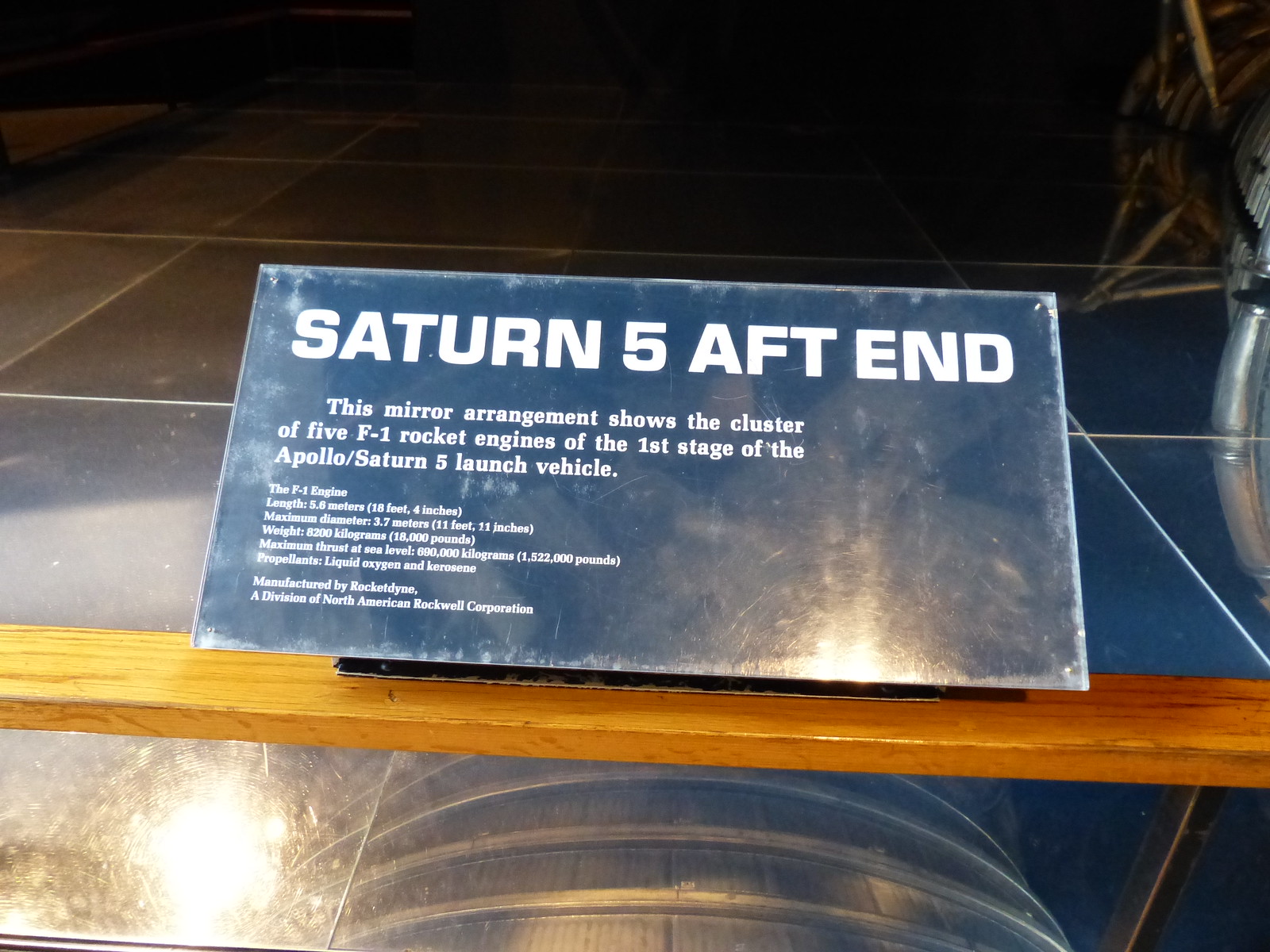This photograph showcases a slightly aged, rectangular blue plaque with white text, mounted on a wooden platform and encased in a plastic protector. The plaque, which looks metallic, possibly aluminum, provides detailed specifications and historical information about the Saturn V rocket's aft end. It states:

"Saturn V Aft End. This mirror arrangement shows the cluster of five F-1 rocket engines of the first stage of the Apollo/Saturn V launch vehicle. The F-1 engine length is 5.6 meters (18 feet 4 inches). Maximum diameter is 3.7 meters (11 feet 11 inches). Weight is 8,200 kilograms (18,000 pounds). Maximum thrust at sea level is 8,000 kilograms-force (1,522,000 pounds-force). Propellants are liquid oxygen and kerosene. Manufactured by Rocketdyne, a division of North American Rockwell Corporation."

The plaque sits atop a reflective surface, possibly mirrors, which enhances the visual presentation of the display. Below the plaque, part of what appears to be a section of the rocket engine, resembling a shaft or tube, is visible. Despite its wear and slight scratches, the plaque remains legible and effectively conveys the impressive details of the Saturn V rocket’s engineering.